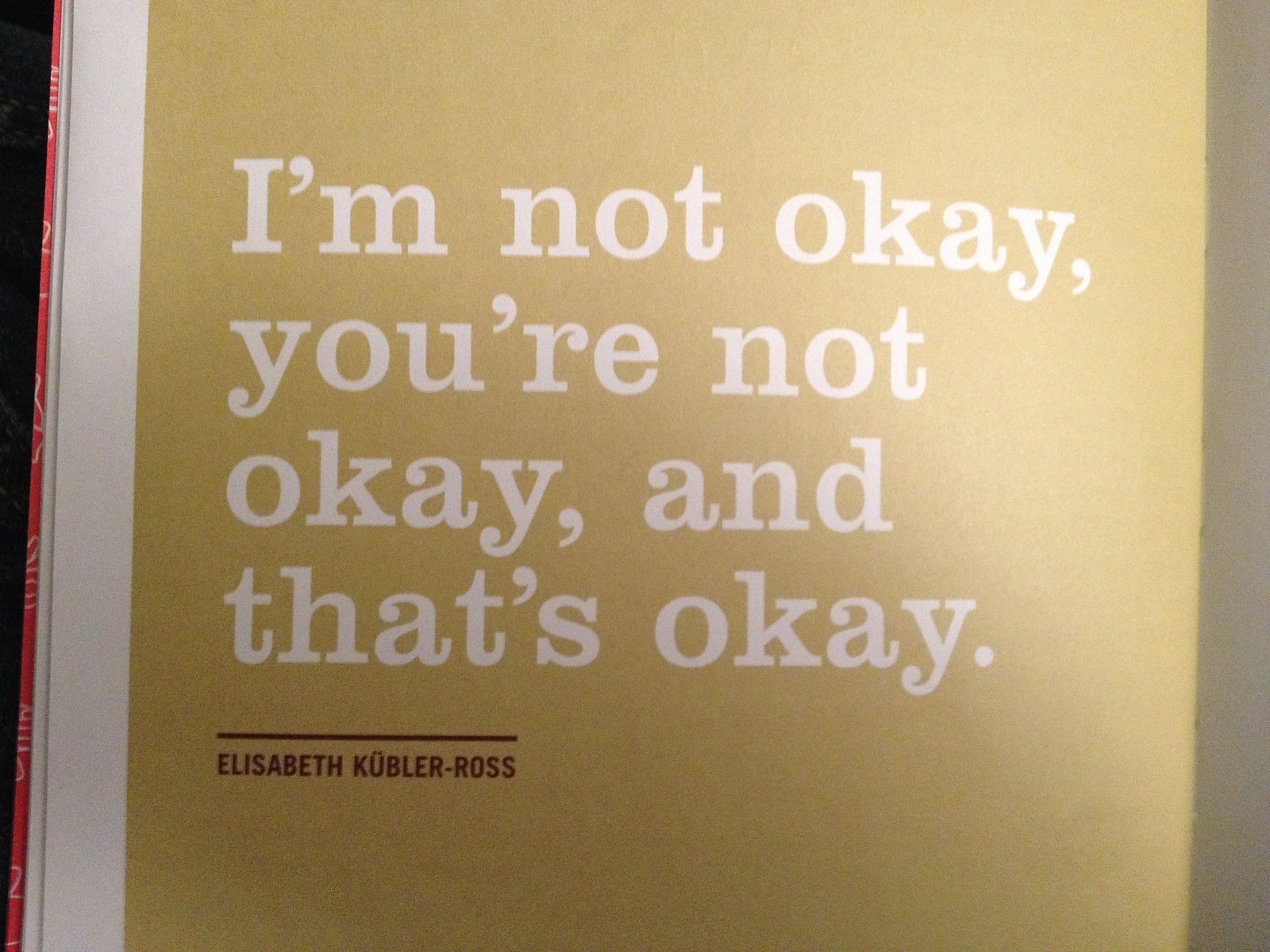The image depicts a page, likely from a book or poster, with a background that varies between a goldenrod or butterscotch color and a beige hue. The text on the page is centralized and prominent, written in large white letters that state, "I'm not okay, you're not okay, and that's okay." Below this, there is a black line followed by the author's name, "Elizabeth Kubler Ross," printed in red. Along the left edge of the page, a vertical red strip is visible, suggesting it could be part of a book cover. The right side of the page shows a shadow or a grayish border. The overall presentation is simple yet striking, with the text in a straightforward font and a minimalistic design.